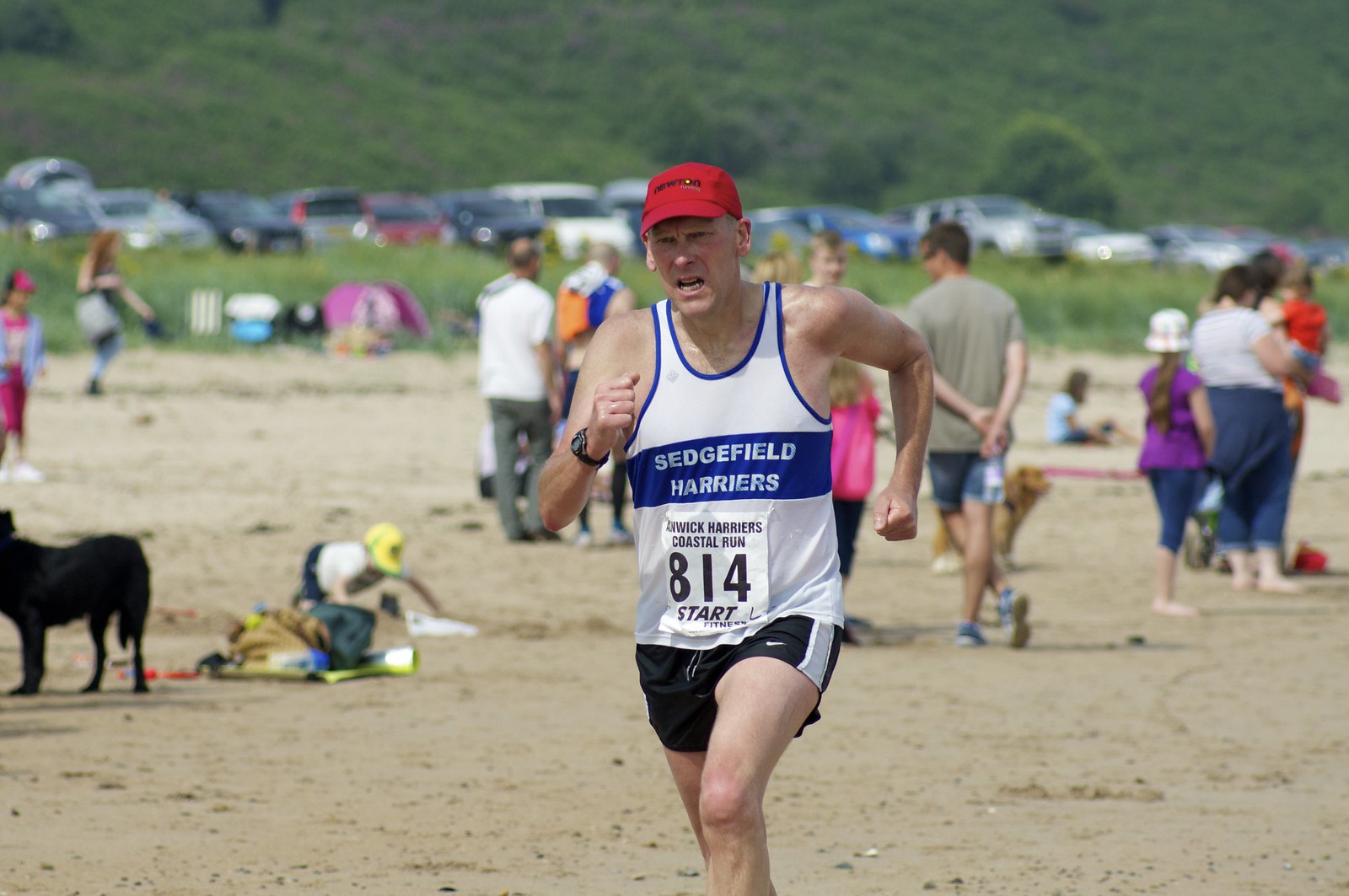This vibrant and dynamic photograph captures an older man running on a busy beach, appearing to be in his fifties or sixties. Wearing a bright red baseball cap, his attire includes a white tank top with blue trim that proudly displays "Sedgefield Harriers" and features a race number "814," hinting at his participation in some sort of competition. His black running shorts are accented with a silver stripe, and on his right wrist, a black waterproof watch is visible. The man's posture, with his left arm pulled back and his right arm forward, suggests he is mid-stride, his fists lightly clenched as he focuses on his run.

In stark contrast to his intense activity, the beach around him is bustling with people casually milling about. Some are dressed in summer attire, ranging from shorts to long pants, neither fully into beachwear. Scattered among the crowd, only a few individuals are seated, possibly accompanied by children. On the far left edge of the frame, a black dog can be seen.

Beyond the sandy beach, a vibrant green hill rises, behind which numerous vehicles are parked. This grassy area at the beach's end suggests an impromptu parking lot or picnic spot, blending into the serene yet lively background. The hill, adorned in green and gray hues, stretches to the top edge of the photograph, slightly blurred, providing a picturesque backdrop to the scene.